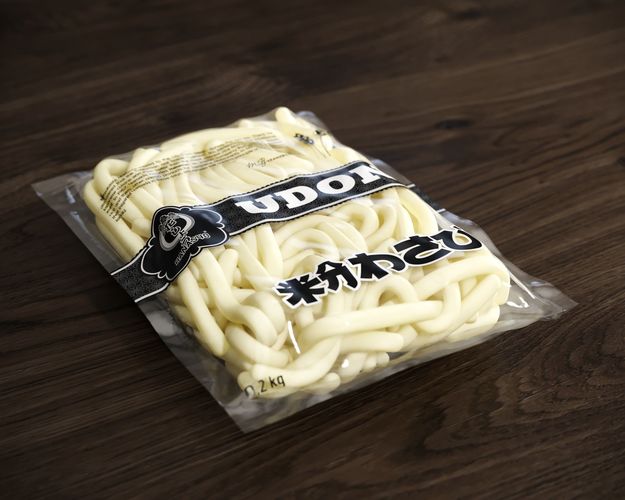This photograph depicts a clear plastic package of udon noodles resting prominently on a brown wooden table. The vacuum-sealed package, with the air removed, showcases the neatly bunched, rectangular-shaped tan noodles visible through the plastic. The central label features the word "UDON" in bold white letters set against a black background, bordered by a delicate black-and-white ribbony design. To the left of the central text is an indistinct company logo, possibly reading "Hanna Sung" or "Hanna Sing," accompanied by a series of black Japanese characters outlined in white. The bottom left corner of the package displays the weight, marked as 0.2 kilograms. The entire scene is captured with the package placed squarely in the center of the image, emphasizing its details against the dark wood grain of the table.